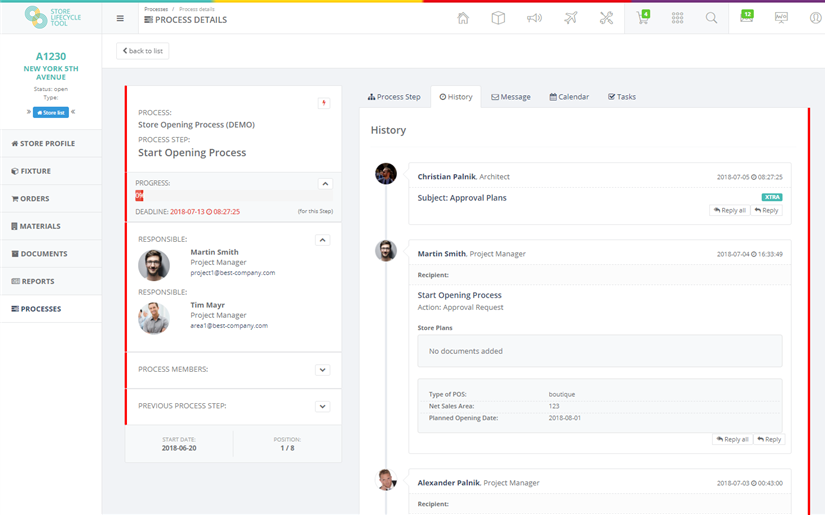This image features a highly detailed process management tool designed for opening a store, displayed on a clean white background. 

**Top Section:**
- **Title Elements:** At the very top, the text "Store Life Cycle Tool" is prominently placed in green on the left side.
- **Process Details:** In black text, the phrase "Process Details" stretches across the top center.
- **Icons:** A row of various icons that visually represent different functions or categories includes a house, a cube, a megaphone, an airplane, a wrench, a shopping cart, and a magnifying glass.

**Left Sidebar:**
- **Store Information:** Displays "A1230, New York, 5th Avenue" with the status marked as "Open".
- **Tabs:** Several functional tabs are listed, including "Store Profile," "Fixture," "Orders," "Materials," "Documents," "Reports," and "Processes."

**Center Panel:**
- **Background:** Features a gray background that’s divided into two columns.
- **Left Column:** 
  - **Process:** Titled "Store Opening Process Demo".
  - **Process Steps:** Lists "Start Opening Process".
  - **Responsible:** Displays Martin Smith and Tim Mayer (spelled M-A-Y-R), both labeled as project managers along with their photos.
- **Right Column:**
  - **History:** 
    - **Christian Palnick:** Architect, subject is "Approval Plans".
    - **Martin Smith:** Project manager, recipient is blank, action is "Approval Request," and no documents are added.
    - **Store Metrics:** "Type of POS: Boutique," "Net sales area: 123".
    - **Important Dates:** "Planned Opening Date: 2018-06-01".
    - **Alexander Palnick:** Project manager, cut-off and not fully readable in the image.

This comprehensive caption explains the intricate layout and details presented in the image, providing a clear and thorough description for better understanding.